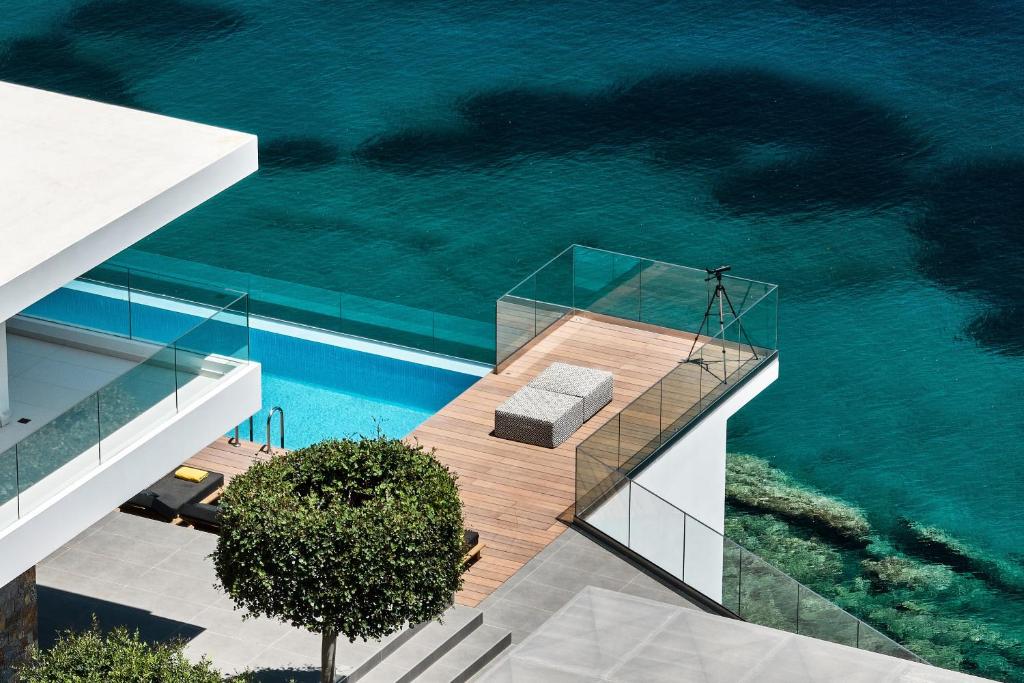This computer-generated aerial image captures a luxurious, modern outdoor setting with incredible detail. It appears to be taken from a drone hovering above a corner of a sleek, upscale house. Central to the scene is a wooden deck featuring a bed in its middle and bordered by short, white glass walls on the edges. Adjacent to the deck, there's a blue swimming pool, bordered by what looks like a wooden slat deck, seamlessly integrated into the patio area. 

On the deck, there is a grey lounge chair positioned near an entrance or ladder into the pool. A significant tree with circularly trimmed leaves is situated in the foreground, adding a touch of greenery to the scene. The deck extends to a glass-roofed structure at its end, enhancing the modern aesthetic. 

To the left, the image showcases part of the modern house with a striking white balcony that features black fencing and rests on a grey floor. This area above the grey lounge chair seamlessly connects to the luxurious design. Below the balcony, a stone walkway interspersed with topiary trees further highlights the opulence of this home. 

In the background, the horizon features a serene expanse of blue and teal water, giving a breathtaking view that epitomizes a high-end, coastal Californian residence. The absence of text in the image allows viewers to fully appreciate the serene, meticulously designed outdoor retreat.